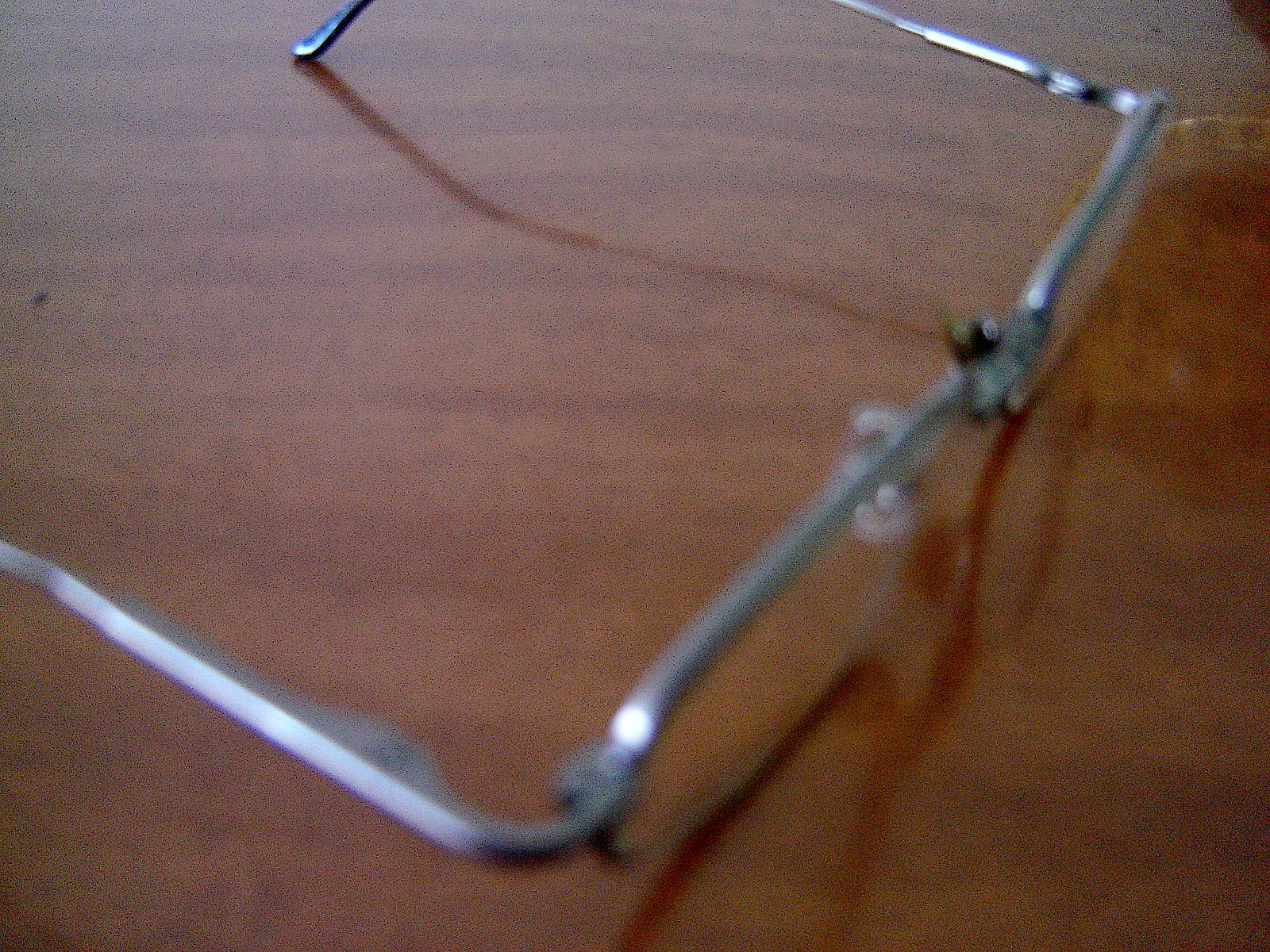A close-up photograph captures a pair of thin, wire-framed, silver-colored glasses resting on a brown wooden table with various shades of brown. The image is slightly out of focus, particularly the lower stems of the glasses which extend towards the upper right of the photo and blur into the background. The table's surface is not shiny, revealing its dull, reddish-brown wood texture. One nose piece on the glasses is silver, while the other displays touches of black and green. The triangular composition shows the left arm of the glasses ending in the upper left-hand corner, in sharp contrast to the completely out-of-focus right arm. The blurry lenses cast shadows on the table, intensified by the light source presumed to be in the upper right-hand corner.